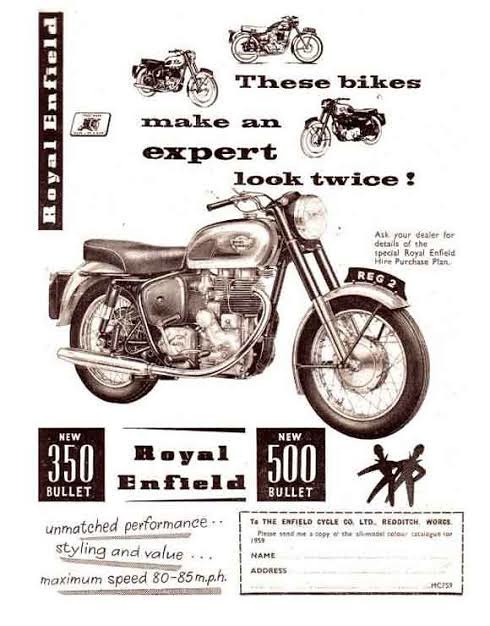The image displays a vintage advertisement for Royal Enfield motorcycles, characterized by a sepia or bronze tint, creating an old-time feel. The central focus is a large graphic of a motorcycle, flanked by three smaller images of different Royal Enfield bikes at the top. The ad is rich with brown and black serif-style fonts, with the striking headline "These bikes make an expert look twice."

On the left-hand side, "Royal Enfield" is prominently displayed. Adjacent to the central motorcycle graphic, the text highlights the special Royal Enfield hire purchase plan with the note, "Ask your dealer for details of the special Royal Enfield hire purchase plan." At the bottom, the ad features the models "New 350 Bullet" and "New 500 Bullet" within designated boxes, emphasizing "unmatched performance, styling and value," and boasting a "maximum speed of 80 to 85 MPH." 

Additionally, there is a small coupon on the lower left side for requesting a catalog, allowing potential customers to fill in their name and address. This meticulously detailed ad uses meticulous typography and layout to attract prospective buyers to the Royal Enfield brand.